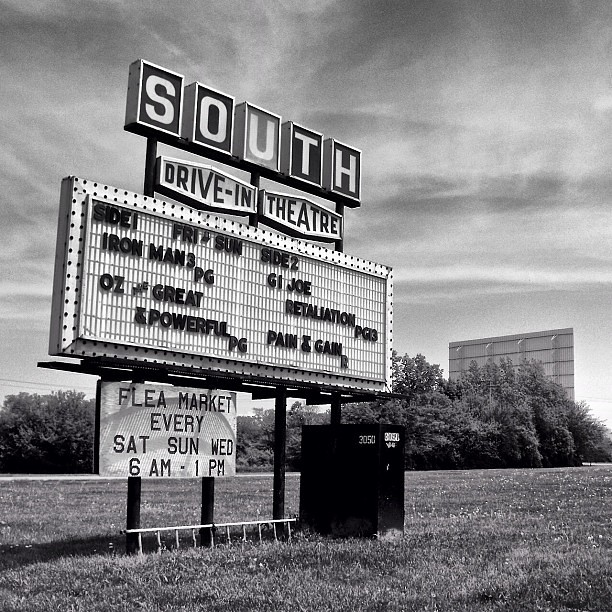This old black and white photograph captures the South Drive-In Theater marquee sign located in the middle of a grassy field. The sky is hazy with some clouds, casting diffuse daylight over the scene. Prominently featured is the marquee, which has adjustable letter tiles and a classic border with decorative dots that likely light up. The sign announces the current movie lineup: on Side 1, "Iron Man 3" (rated PG) and on Side 2, "Oz the Great and Powerful" (rated PG) along with "G.I. Joe Retaliation" (rated PG-13) and "Pain and Gain" (rated R). Below these listings, a smaller sign advertises a flea market happening every Saturday, Sunday, and Wednesday from 6 a.m. to 1 p.m. At the base of the marquee, there's a ladder lying on its side and a black transformer box with the number 3050 visible in the upper right corner. The background is filled with trees, which add to the nostalgic atmosphere of the drive-in theater.